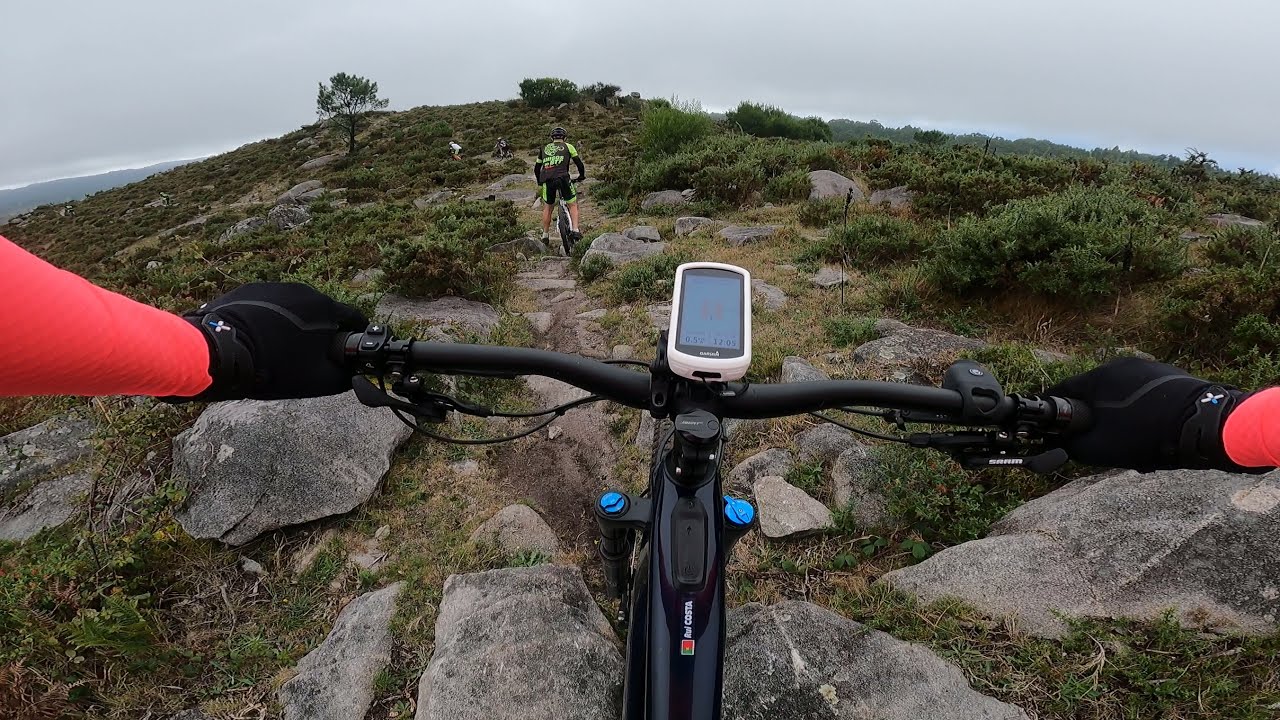The photograph captures the perspective of an individual mountain biking on a rugged, rocky trail. The black and blue mountain bike they are riding is partially visible, with black handlebars firmly gripped by hands clad in black gloves. The rider is wearing a distinctive long-sleeve, bright red or slightly orange-red shirt. A white GPS tracker is mounted at the center of the bike's frame. Ahead on the rocky path, another biker, dressed in black and neon green attire, rides a white mountain bike. The trail is surrounded by low green bushes, grass, and various foliage, with numerous boulders scattered around. A single tree stands slightly to the left center of the image. The background also reveals several other bikers further along the path. The sky overhead is a solid gray, giving the scene a misty, overcast ambiance, with no hint of sunlight.